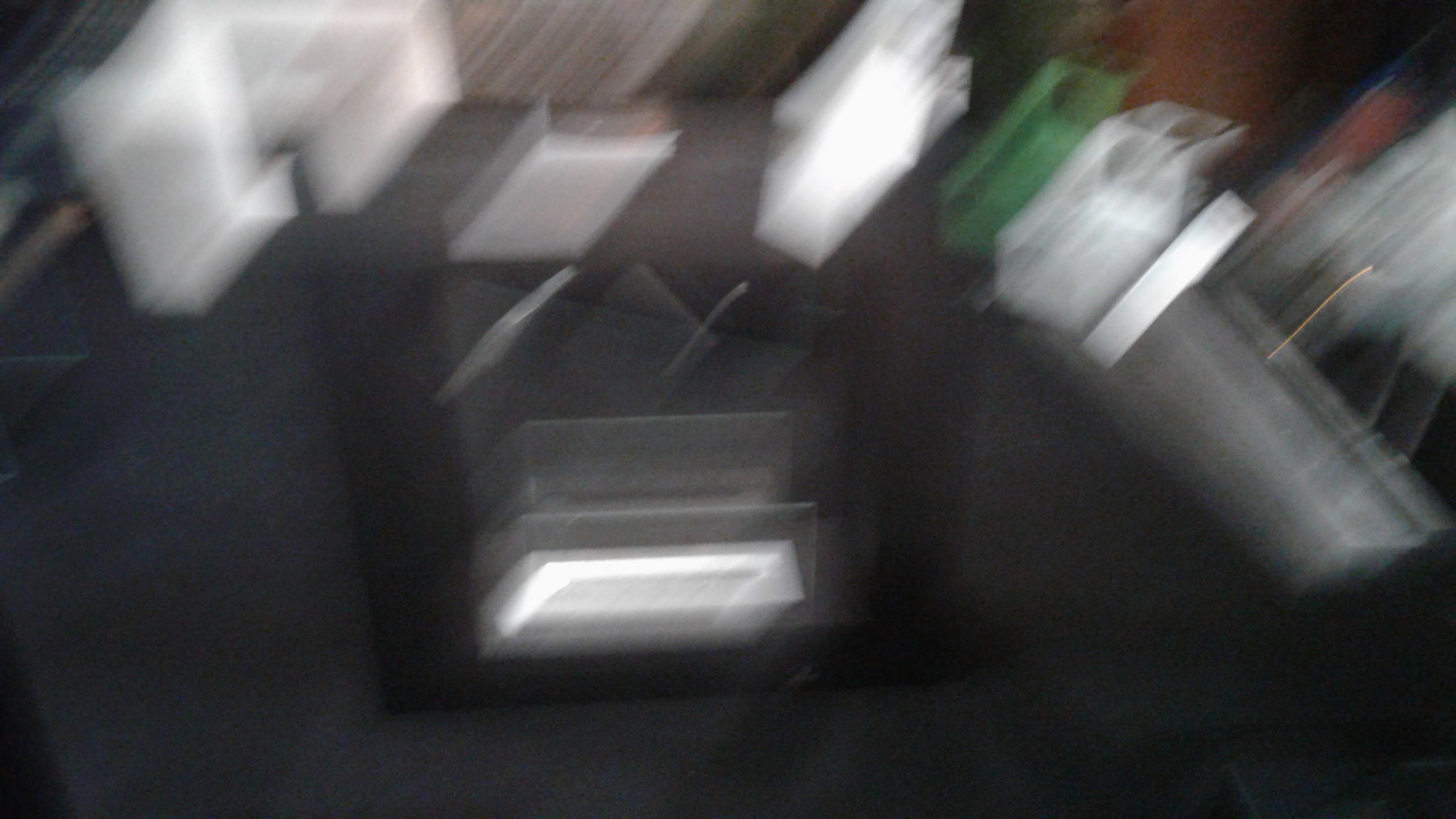The photograph is extremely blurry, making it difficult to identify specific objects with certainty. The scene appears to be in motion, contributing to the distorted and transparent appearance of several shapes. Dominating the image are a series of recurring blurred, semi-rectangular and square forms, with circles embedded in some of them. Significant objects include a green rectangle that features a circle, a central black box adorned with white rectangles hanging off its sides, and several small black boxes with diverse silhouettes scattered across the scene. These shapes and boxes repeat throughout the image, adding to the sense of motion and distortion. In the background, a red box with a blue lining is faintly visible on the right side, further adding to the complexity of the composition. The overall effect is one of chaotic, abstract movement, primarily defined by its unclear and overlapping forms which might suggest office supplies but remain indistinct due to the blurriness.